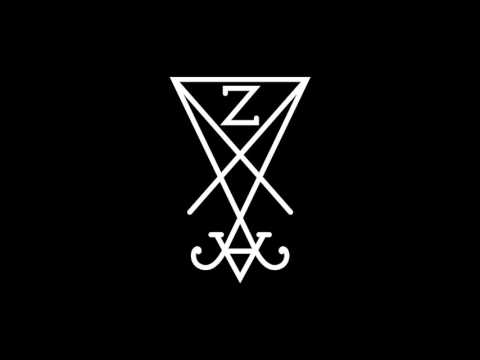The image features a stark black background, prominently showcasing a white geometric design. At the center lies an intricate upside-down triangle, which contains a smaller upside-down triangle within it. The apex of these nested triangles extends upward, and inside the smaller triangle, a bold white letter "Z" is prominently displayed. Beneath the larger triangle, a shape resembling an upside-down "A" or "V" is present, accompanied by two elegant curly lines that spiral outward from its base. The entire composition is composed of straight white lines with a few curves, creating a striking and elaborate design against the dark backdrop. The exact purpose of the image is ambiguous, potentially serving as a stylized logo or an abstract artistic design.